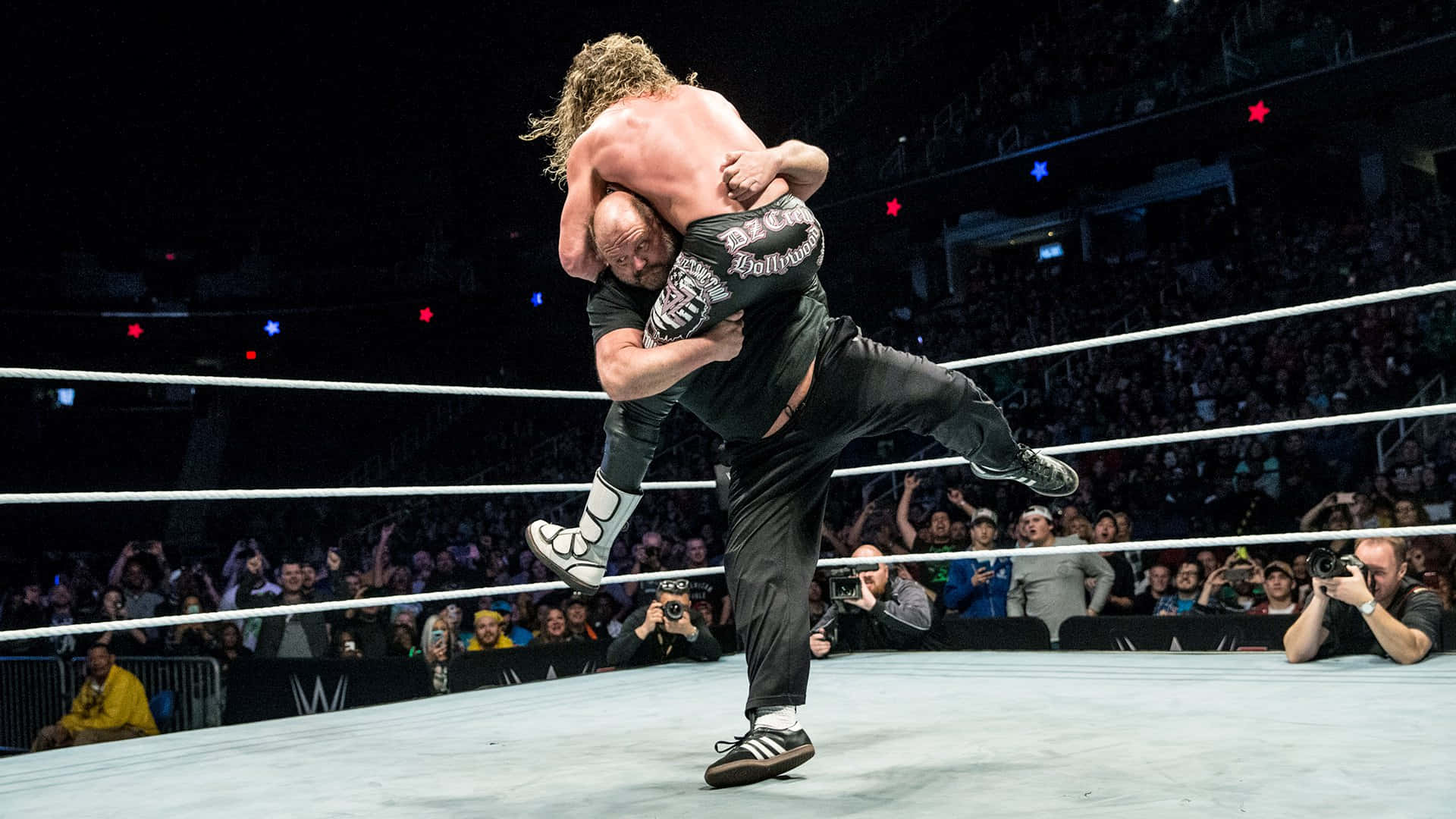In this dynamic WWE wrestling match scene, the action is centered in a traditional wrestling ring with white ropes and a gray mat. The background is dark, making the brightly lit ring the focal point. Blue and red lights add dramatic flair, shining down around the ring, emphasizing the spectacle. Surrounding the ring is a packed audience, their cheers filling the air, and among them are security personnel and cameramen capturing the electrifying moment. In the ring, a larger wrestler in a black t-shirt, black pants, and Adidas sneakers is lifting his muscular, shirtless opponent who has long blonde hair and wears black pants emblazoned with "DZ Hollywood" on the back paired with white designer boots. The shirts-off wrestler is about to be slammed onto the mat, creating palpable tension in the arena. WWE logos can be seen on the barricades, underscoring the event’s grandeur.